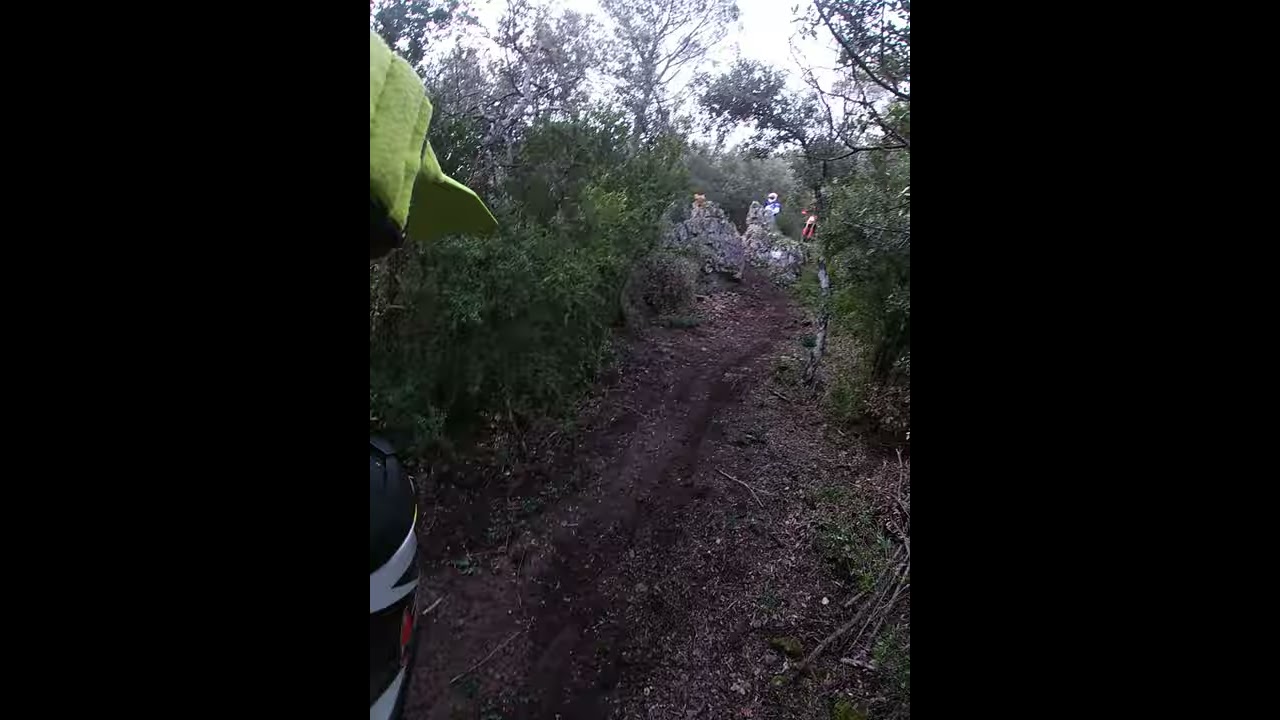The photograph captures a dirt path cutting through dense greenery, probably taken from a first-person perspective, possibly using a GoPro camera. The scene is set during daytime under a white, sunlit but overcast sky, casting a well-lit but softened light over the surroundings. The path, naturally formed and brown with a few darker streaks from bike tracks, extends from the bottom left toward the center of the image. It is flanked by thick brush, green trees, and shrubs, along with twigs and mulched leaves scattered on the ground.

In the distance, partially obscured by the foliage, stand several individuals. One appears to be wearing a motocross outfit with a helmet, accompanied by a bike, likely atop a rocky structure. Another person in a red outfit and one in a white outfit can also be discerned. Near the left edge of the image, there is a partial view of another biker or their bike, with only an arm and the bike's details visible. The foliage is dense but becomes sporadic near the top, allowing glimpses of the cloudy, off-white sky. Vertical thick black strips frame the left and right side of the image.